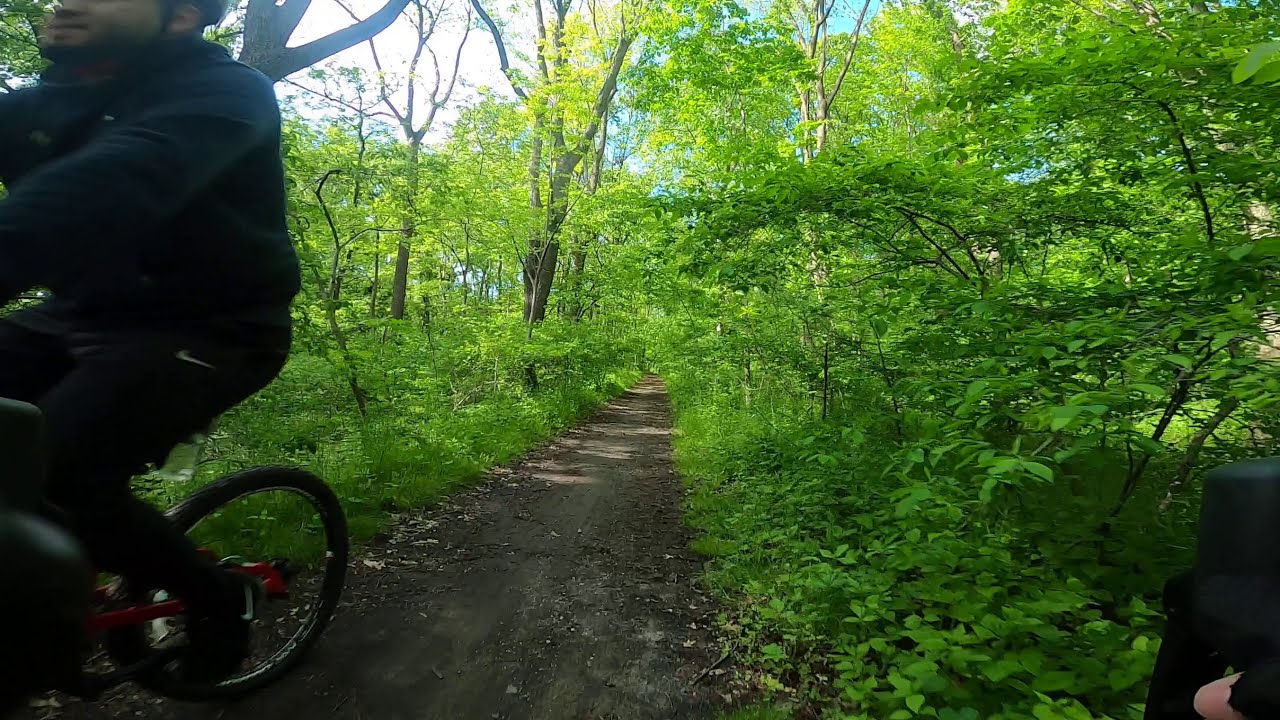The photograph captures a vivid outdoor scene on a bright, clear day with a blue sky and scattered white clouds. Central to the image, a well-trodden dirt path begins from the lower center, extends to the left, and curves inward, leading the viewer's eye towards the midline. On the left side of the path, partially cropped out by the frame, a bicyclist with brown skin is riding a red bike. He is wearing a black long-sleeve shirt, black pants featuring a white Nike logo by the pocket, and a black helmet, though the top half of his head is cut off by the photograph's edge. The motion blur suggests he is riding at a decent speed. 

Surrounding the path, a thick, lush tapestry of green trees and foliage frames the scene, indicating a springtime setting with the fresh, vibrant green hues of newly sprouted leaves. The right-hand side of the image also includes a partial view of a Caucasian person's finger, holding a black thermos in the bottom right corner. The overall composition balances human activity with the tranquil beauty of nature.